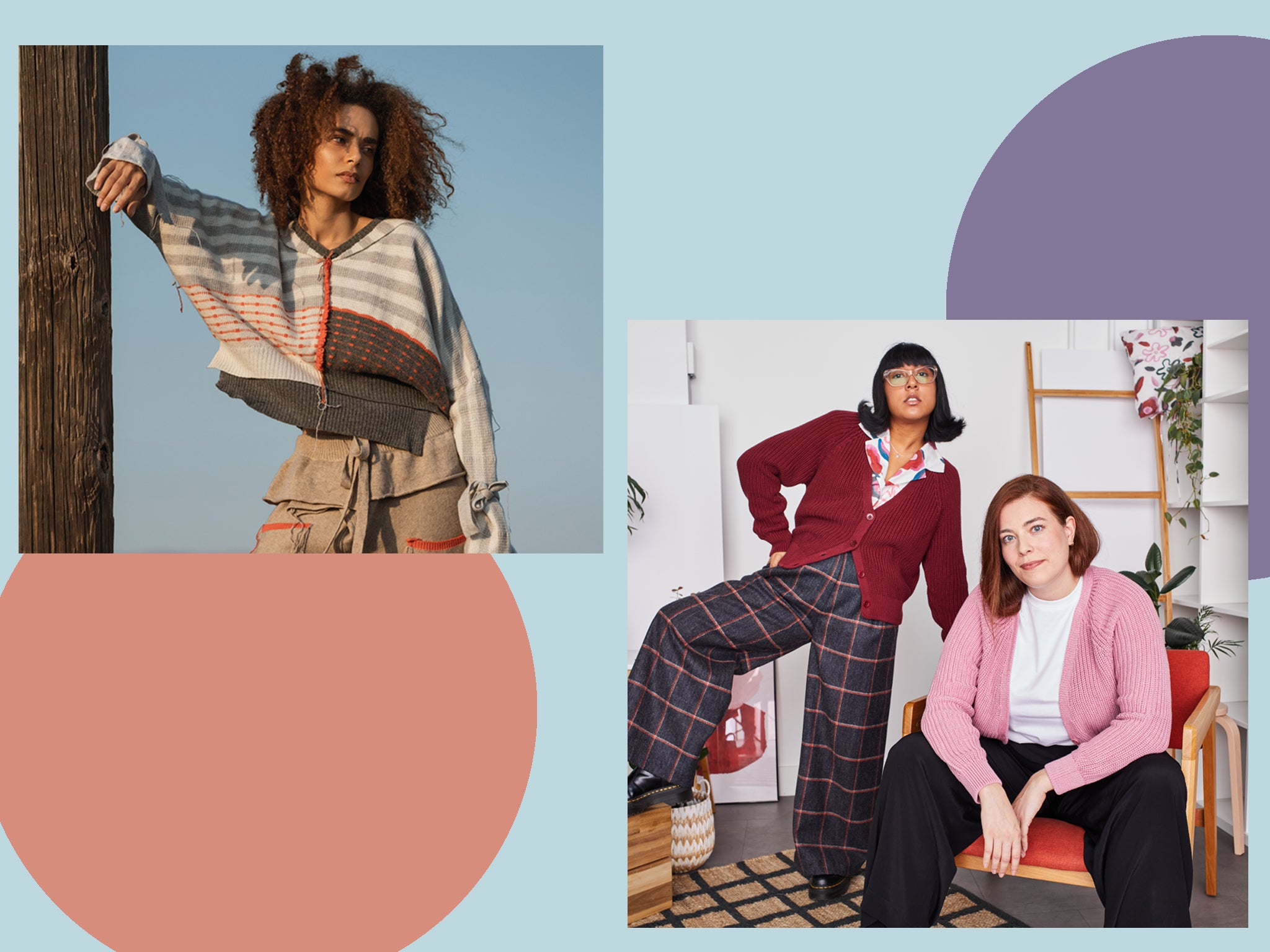The collage features two distinct photographs set against a light blue backdrop with an artistic touch. At the bottom left, there is a large, vibrant orange circle, while the top right houses a partial light purple circle. 

In the top left corner of the collage is a square photograph capturing a serene moment. Against a clear blue sky, a woman stands facing the camera with her head slightly turned away. She has shoulder-length, extremely coily and curly dark hair and medium tan skin. Her right arm is casually resting against a wooden post, adding a relaxed vibe to the scene.

The bottom right corner of the collage showcases another photograph, this time indoors. Two women are prominently featured. The woman seated in a red chair is dressed in black pants and a white shirt layered with a pink ribbed sweater. She has chin-length red hair. Beside her stands another woman with one leg propped on a wooden box. She wears dark plaid pants, a red cardigan, and a white collared shirt with a pattern. Her black hair is complemented by glasses, adding to her distinguished appearance.